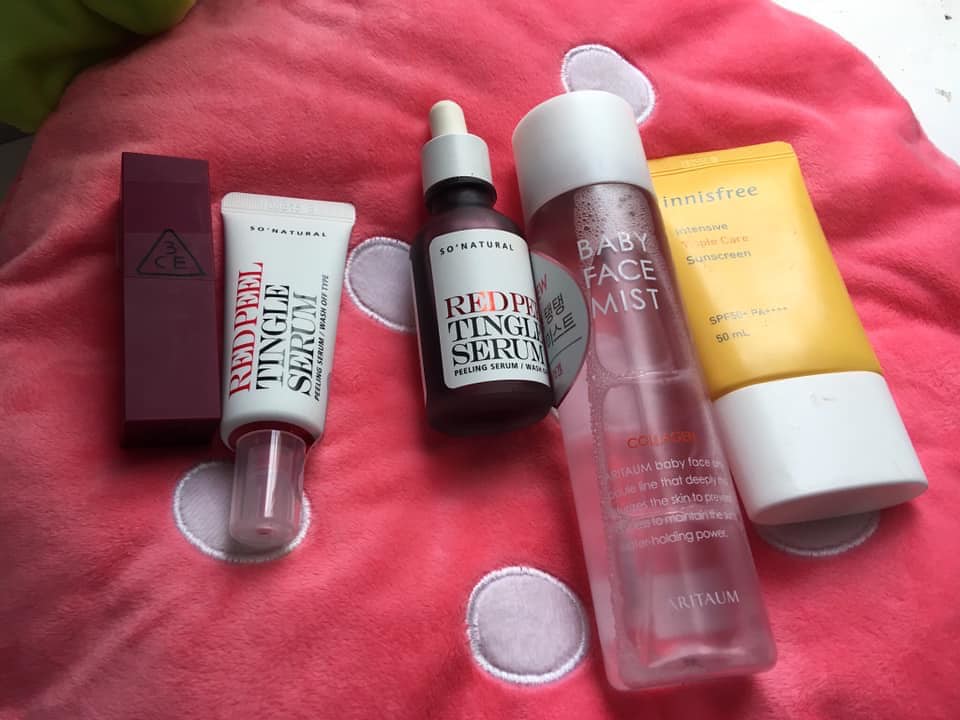The photograph showcases an array of beauty and skincare products meticulously arranged on a pink pillow adorned with white polka dots, resembling a strawberry complete with a green portion at the top (partially cropped out of the image). On the left side, there is a sequence of four distinct products neatly aligned. The far left features a maroon-colored box branded with "3CE." Adjacent to it is a white tube capped with a clear lid, labeled "Red Peel Tingle Serum, Peeling Serum, Wash Off Type." Following that is a maroon bottle with a white dropper-style lid, bearing the "So Natural, Red Peel Tingle Serum" designation. The lineup concludes with a larger, clear bottle capped in white, and labeled "Baby Face Mist Collagen" with additional indescribable text at the bottom. To the right of this lineup is a yellow container, a tube with a white cap at the bottom, prominently marked with "INNISFREE, Intensive Tropic Care Sunscreen, SPF 50, 50 ml."